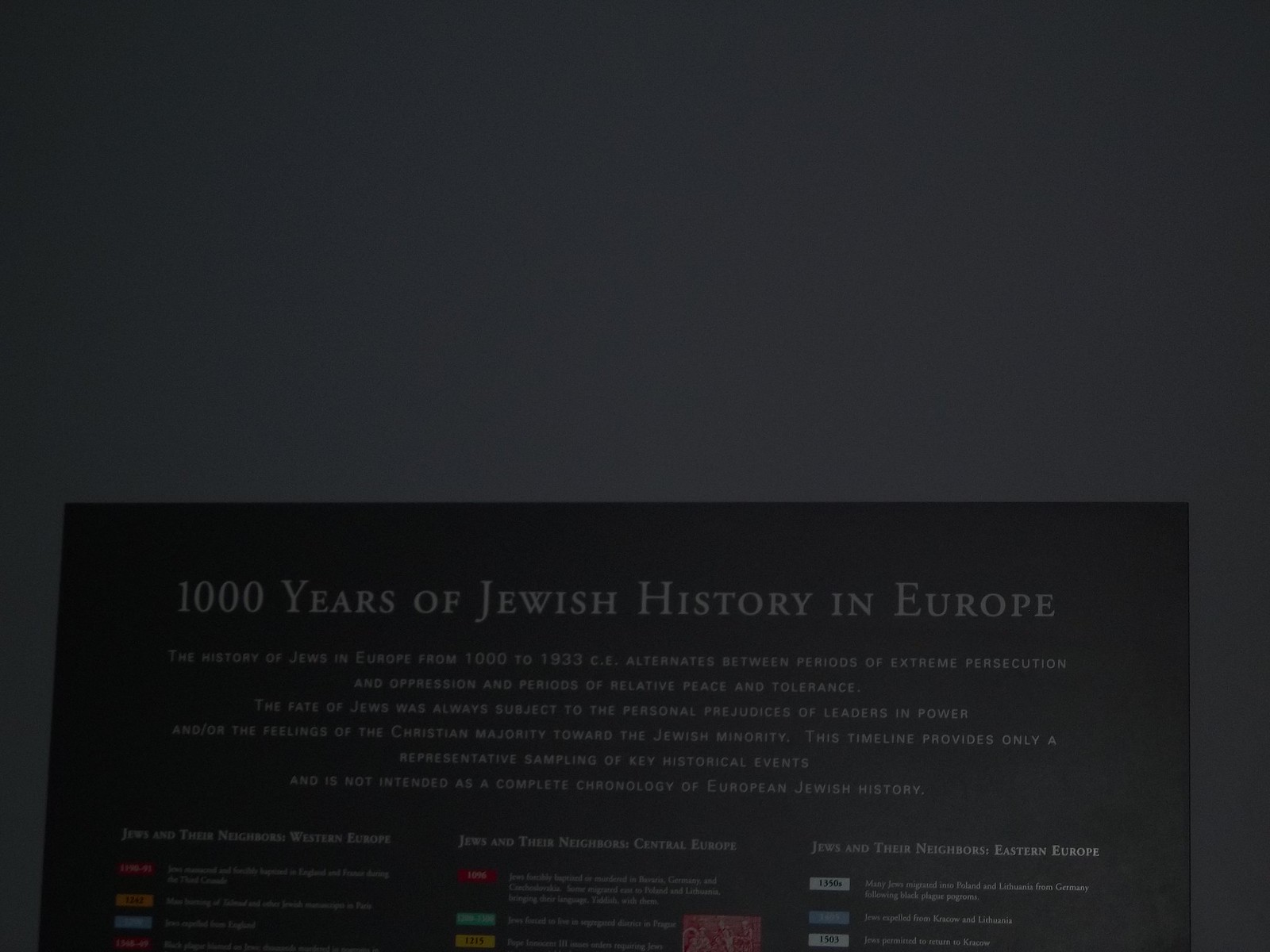The image depicts a widescreen photograph of a dark, smooth, and deep gray wall, with a partially visible sign at the bottom. The sign, almost spanning the width of the image, features a black background with gray text that reads "1,000 years of Jewish history in Europe" at the top. Below this title, in smaller all-capital gray letters, the sign describes the varying experiences of Jews in Europe from 1000 to 1933 CE, alternating between persecution and periods of relative peace. It notes that Jewish fate often hinged on the prejudices of leaders and Christian majority sentiments, and the text then mentions that the timeline provides a sampling of key events, not a complete history. Beneath this explanatory text, there are three columns with additional historical details, accompanied by small colored icons in hues of red, orange, green, yellow, and gray, though the specifics of these sections are too small to be clearly readable.